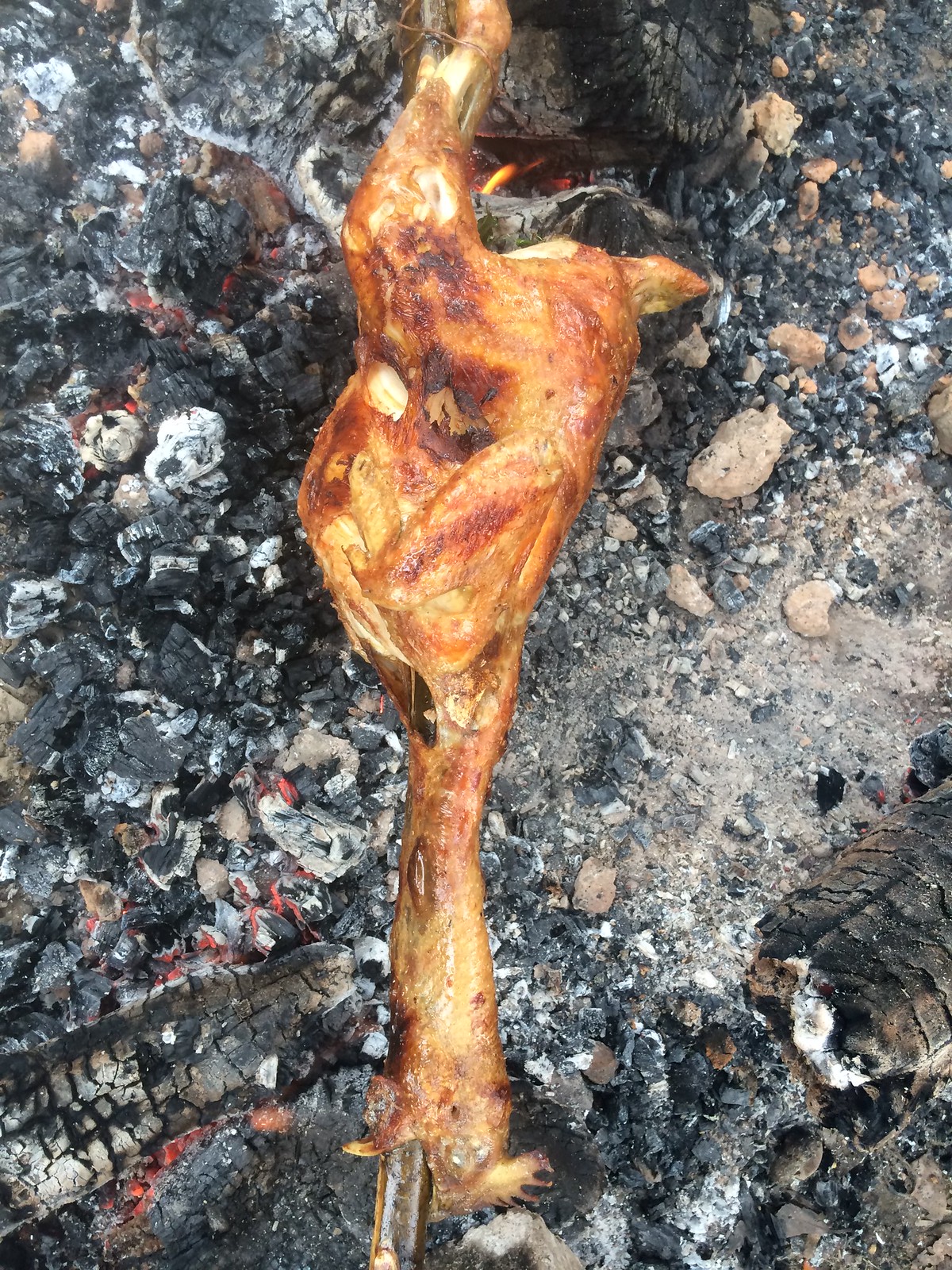The photograph features a vertically aligned, rectangular image with a focal point on a roasted piece of meat. The background is a dense mix of speckled charcoal, rocks, and glowing embers in shades of black, gray, brown, and bright red. The central object appears to be a skewered whole chicken, from head to tail, prominently displayed from top to bottom. The chicken has been coated with barbecue sauce, giving parts of it a dark brown, almost reddish hue. It is evident that the meat has been roasted, exhibiting a golden color in some areas and a darker brown in others. The setup suggests that the chicken is either on a rotisserie or lying directly on a bed of coals, implying an outdoor cooking environment, perhaps a campfire rather than a traditional grill.